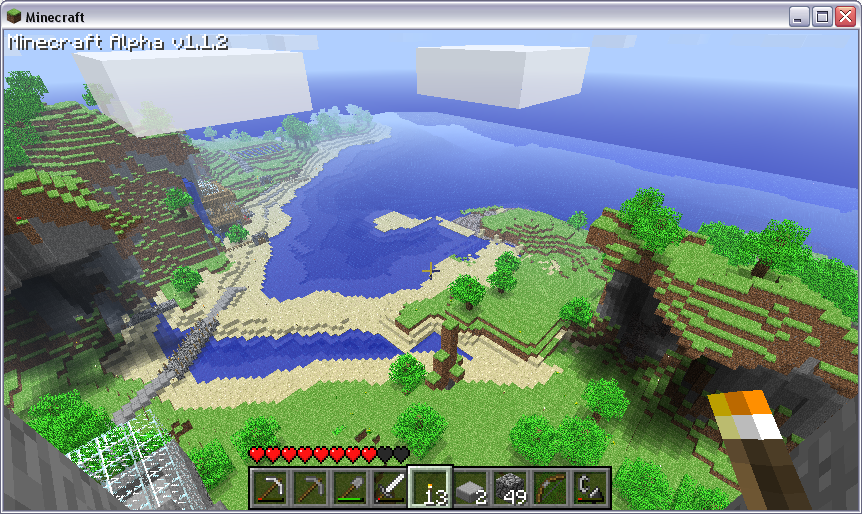A screenshot captured from the alpha version 1.12 of the popular video game Minecraft. The landscape features a serene beach adjacent to rolling grassy knolls dotted with blocky, pixelated trees rendered in the characteristic 8-bit or 16-bit style. Towering cliffs rise in the distance, while large, square clouds float across the sky, adhering to the game's iconic, simplistic aesthetic. The player is missing two hearts from their health bar, visible at the top of the screen, indicating some recent damage taken. Additionally, a prominent red X is noticeable in the upper right corner, likely signifying a system or interface message.